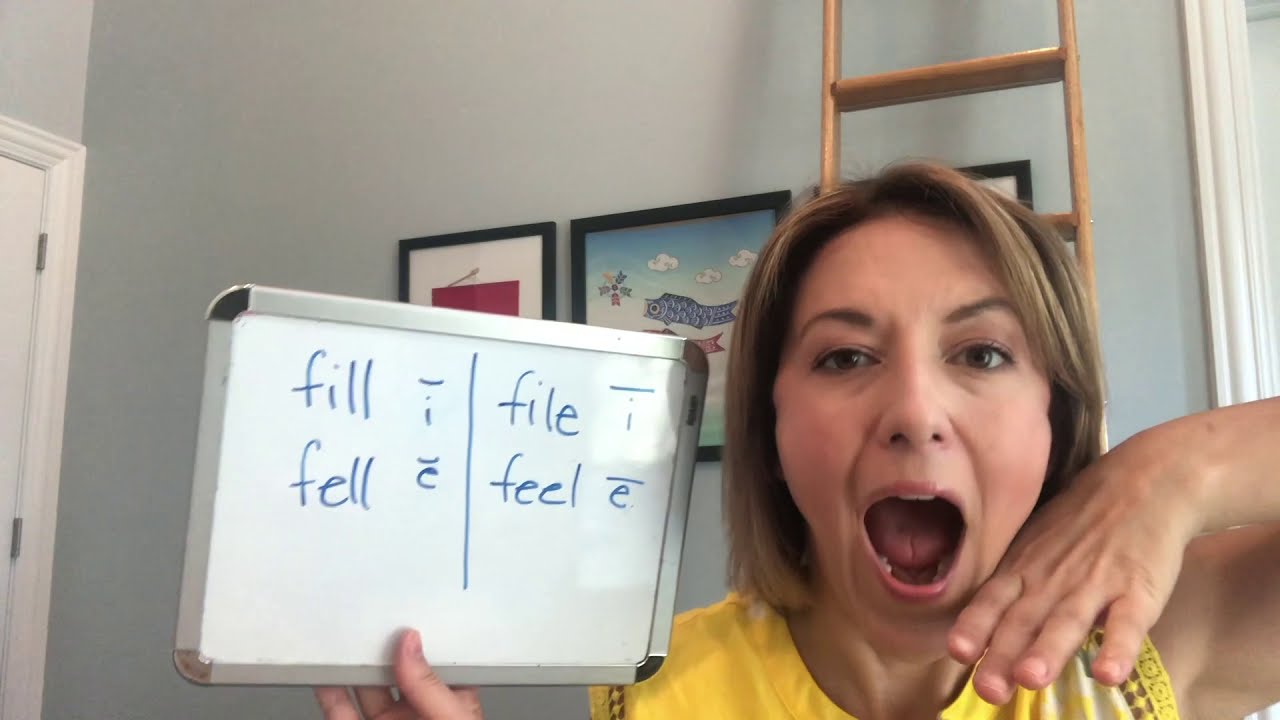The image shows a woman with light skin and short, dirty blonde hair, wearing a sleeveless yellow shirt, positioned in the bottom right corner of the frame. She appears to be teaching pronunciation, her mouth open wide as if enunciating words. She holds a small whiteboard with a silver border in her left hand. The board features four words written in blue: FILL, FELL, FILE, and FEEL. To aid in pronunciation, there is a line above the I in FILL, a line below the E in FELL, a line above the E in FEEL, and a line above the I in FILE. The background reveals a home or office setting with a light blue wall, a white door with decorative molding, a brown wooden ladder, and three framed photos. The left image in the frames shows a white scene with a red square, the middle one depicts a sky with fish, and the third is partially obscured.